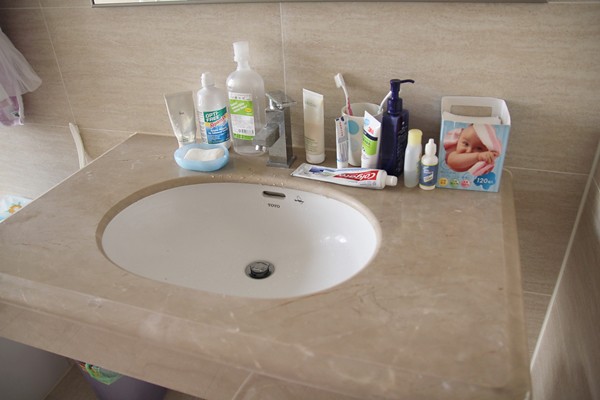A detailed depiction of a bathroom sink area:

The sink has a beige marble finish with variations of white streaks. To the right of the sink, there is a package featuring a photograph of a baby wrapped in a pink hooded towel bordered with white. Adjacent to the package on the left, there is a small bottle resembling eardrops or eye drops. Positioned next to that is a small container of baby shampoo or soap.

Moving further left, there is a long, rectangular dark blue bottle. It has a wide base that narrows towards the top and features a thick spout with a thin, narrow outlet for dispensing lotion or soap. Besides this bottle, there is a tube adorned with pink and blue shapes, which is positioned behind a used Colgate toothpaste tube resting at the front.

Within the basin, the drain stopper exhibits a traditional metal color. The sink basin itself, likely made of porcelain, is white. On the left side of the image, a lacy towel or washcloth with white and pink patterns is hanging up.

The background wall behind the sink is beige with medium brown brush stroke patterns and hints of white that complement the sink's color scheme.